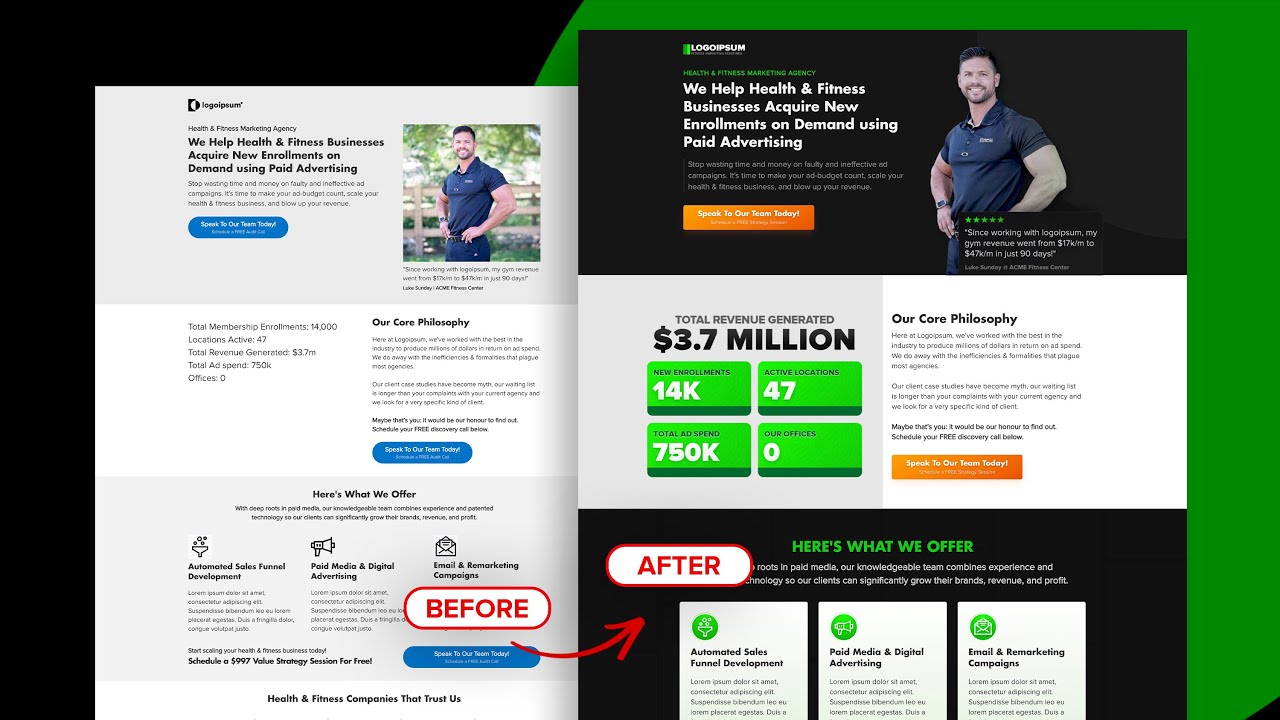The image displays a before-and-after comparison of a website redesign set against a black background featuring a green elliptical shape occupying approximately two-thirds of the background. The top left third of the image remains black, while the green spans the remaining area with a slight touch of black in the bottom right corner. 

**Before (Left Side):**
The original website design is segmented into three horizontal sections: a grey block at the top, a white middle section, and another grey block at the bottom. 

- **Top Section:** This section features a photograph placed on the top right, accompanied by descriptive text on the left and a prominent blue button.
- **Middle Section:** On the left, there's some text followed by significant white space, and a paragraph aligned on the right with another blue button beneath it.
- **Bottom Section:** This grey block is divided into three columns, each containing an icon at the top with relevant information listed below.

A word "BEFORE" is overlayed on this side with a red curved arrow pointing towards the new site on the right side.

**After (Right Side):**
The redesigned website retains the three-section layout with some changes in background colors and content arrangement:

- **Top Section:** The top and bottom sections now feature a black background. The middle section is split into a grey left half and a white right half.
  - The photograph of a smiling white man with a moustache and goatee, wearing a short-sleeved blue t-shirt with his hands on his hips, has been edited to remove the background. A review is added on top of this picture. To the left of the photograph, the name of the site is prominently displayed, followed by a headline stating, “We help health and fitness businesses acquire new enrolments on demand using paid advertising.” Additional details are provided in small print accompanied by an orange button below.
- **Middle Section:** The left grey half highlights the total revenue generated ($3.7 million) along with four green blocks containing white text and some black headlines. The right white half presents the core philosophy of the business as the headline, with a detailed paragraph below it and another orange box for checking some options.
- **Bottom Section:** This section features a black background with a green headline, "Here's what we offer," followed by white text. The three columns now contain three white blocks, each with an icon in the top left corner, followed by a headline and detailed information.

The transformation emphasizes a modernized, user-friendly, and visually engaging design, enhancing both functionality and aesthetic appeal.